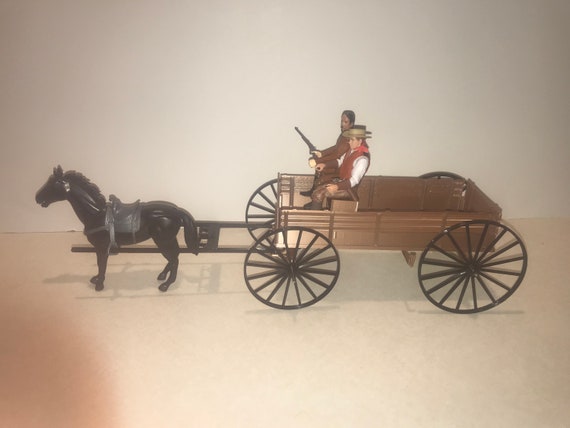The photograph captures a detailed toy setup featuring a small black horse with a gray saddle, pulling a brown wagon with large black wheels. The scene is laid out on a white surface with a white background, and there appears to be a shadow from the person taking the picture. The horse, positioned in the front left of the image, is accompanied by two detailed figurines. The first figurine, an Indian dressed entirely in brown and holding a pistol, sits to the right. The second figurine, a cowboy wearing a beige cowboy hat, a brown vest, a white shirt, and dark pants, stands on the left. The cowboy figures as if he's in control of the horse, although no reins are visible. Notably, the bottom left corner of the photograph is partially obscured by a finger, adding an unintended personal touch to the image. This scene vividly brings to life a miniature Western tableau.